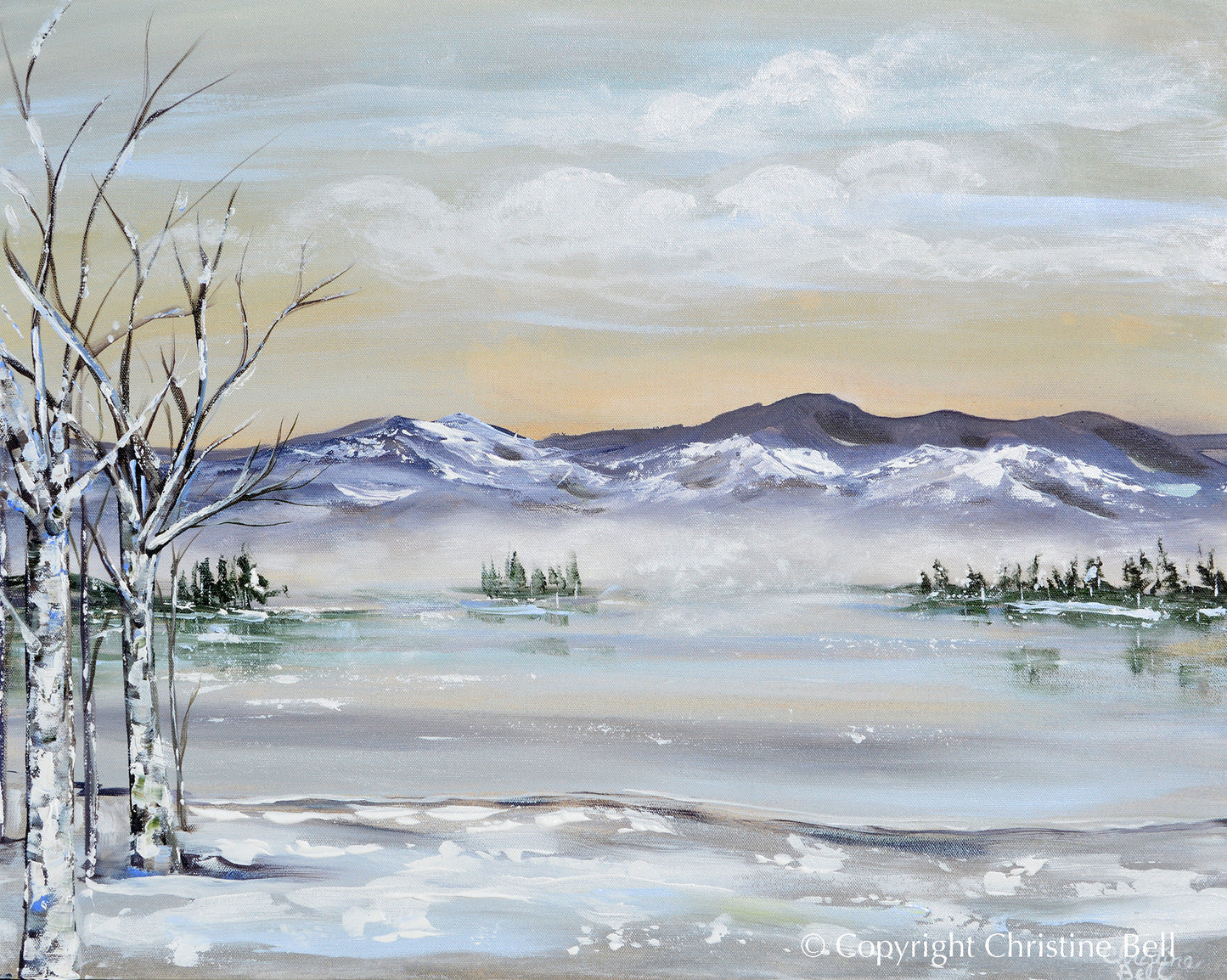This painting by Christine Pell depicts a stark and serene winter scene characterized by its extensive use of pastels in pinks, blues, and whites. The central focus is a frozen lake, rendered in shades of gray, blue, and beige, which mirrors the overcast sky above. The sky itself is a gradient of gray with hints of pink, light blue, and yellow, suggesting an imminent snowfall. Surrounding the lake are snow-capped mountains in the distance and clusters of barren trees with silvery bark, particularly prominent in the left-hand corner. The ground beneath these trees is a snowy white hill, adding to the overall chilly ambiance. The painting captures the quiet, cold beauty of winter, with textured, fluffy clouds adding depth to the scene. The signature "Copyright Christine Pell" can be found in the bottom right corner, confirming her distinctive artistic style.